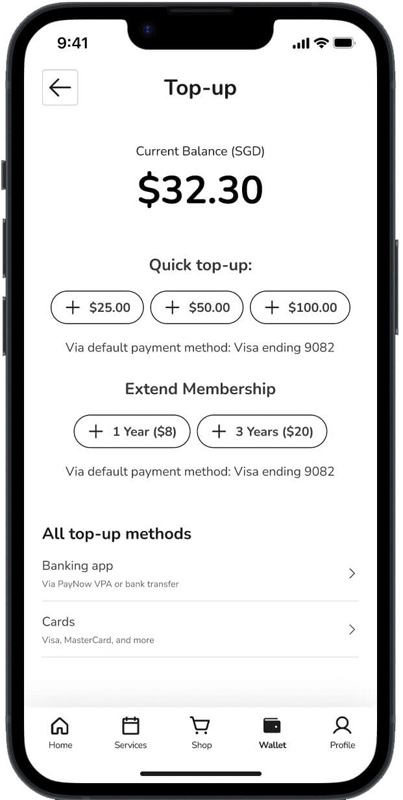The image depicts a smartphone screen with various details visible. At the very top left corner, the time is displayed as 9:41 AM. On the top right, there are icons indicating cellular signal strength, Wi-Fi connectivity, and a nearly full battery symbol. Directly below these status icons, the large header "Top-Up" is prominently displayed.

On the top left side of the screen, there's a backward-pointing arrow encased in a gray square outline. Centered beneath "Top-Up," the text "Current Balance" is shown with "SGD" in parentheses. This is immediately followed by a display of the current balance, which reads $32.30.

Further down, the section titled "Quick Top-Up" offers three selectable options for topping up the balance: $25, $50, and $100. Beneath these options, the text indicates the default payment method as "Visa ending in 9082."

Subsequently, there's a section allowing users to extend their membership. Options here include extending for one year at $8 or three years at $20, both payable via the same default Visa card ending in 9082.

The "All Top-Up Methods" section follows, listing the options of using a banking app or cards, with the latter positioned just below the banking app option.

At the bottom of the screen, there are five icons spaced evenly across the screen, labeled "Home," "Services," "Shop," "Wallet," and "Profile," respectively.

The smartphone itself is encased in a black border on all four sides, framing the entirety of this detailed interface.